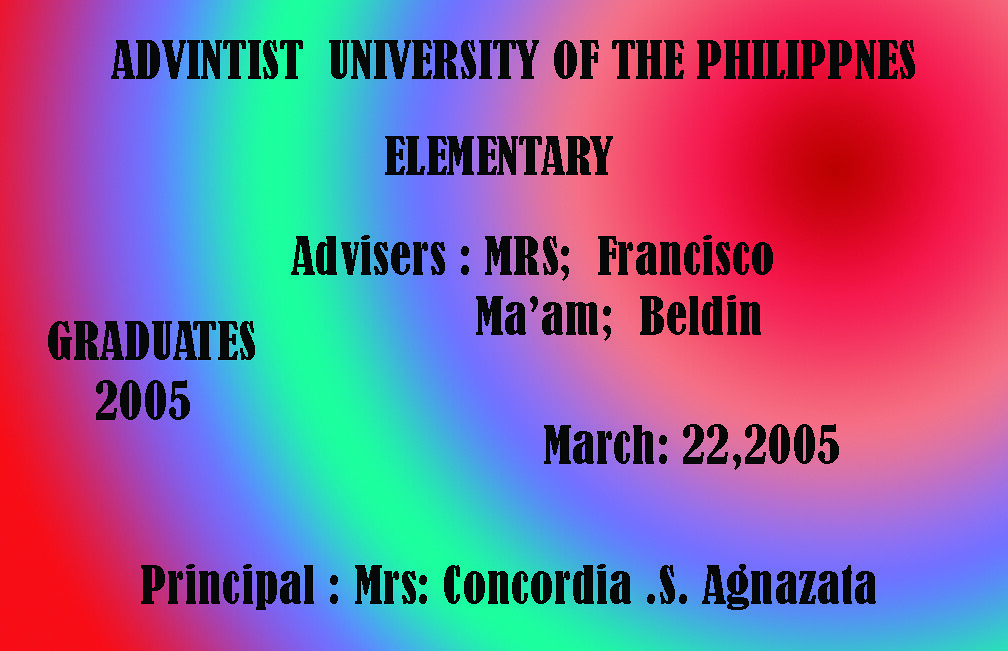This image features text and a vibrant, colorful background. The text, written in black letters, is positioned at the top and reads: "Adventist University of the Philippines Elementary Advisors: Mrs. Francisco and Ma'am Belden. Graduates 2005, March 22, 2005. Principal: Ms. Concordia S. Agnes Ata." The background consists of multiple colored concentric circles, transitioning smoothly from one color to another, starting with a lighter red that darkens into orange, then transitioning to pink, purple, blue, green, and back to variations of blue, purple, pink, and red. These circles span from one side of the image to the other, creating a visually engaging gradient effect. This appears to be a school-related announcement or advertisement, possibly a directory or pamphlet, celebrating elementary school graduates.